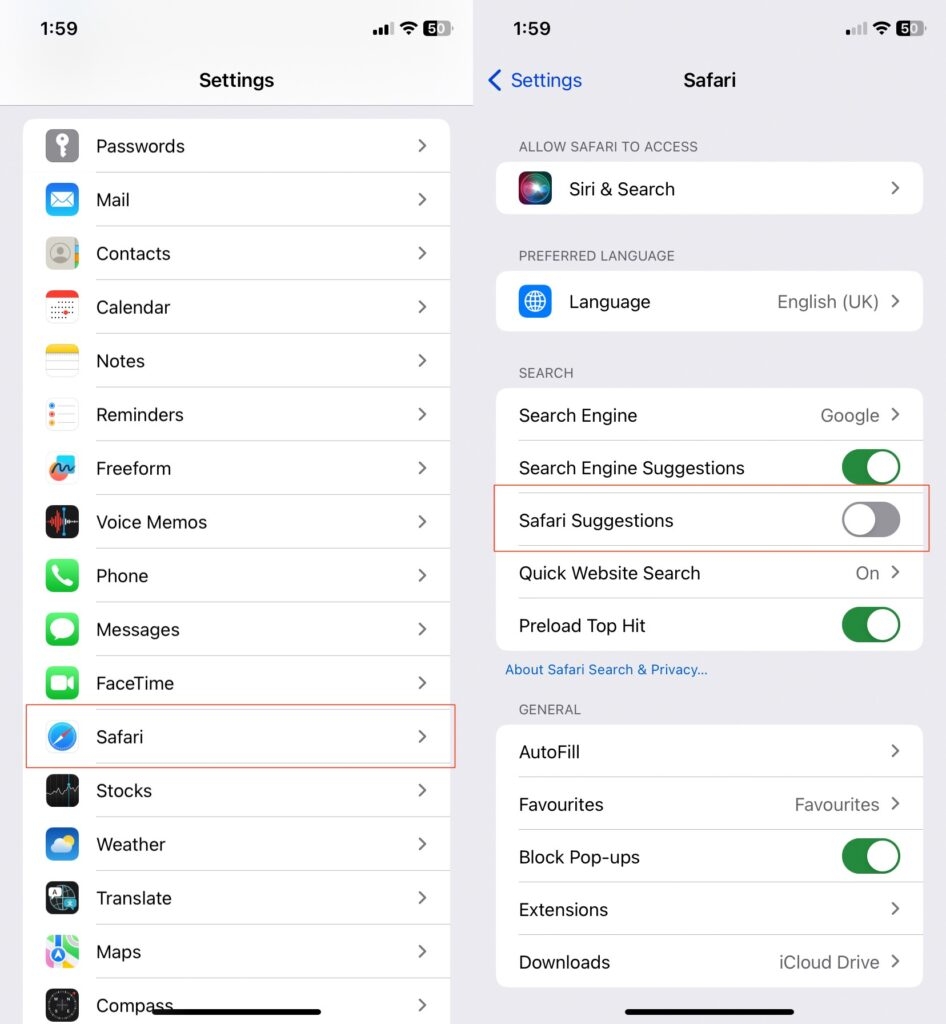This image captures a smartphone screen displaying two adjacent screenshots with detailed settings menus. The top bar of the smartphone screen shows the time as 1:59, along with icons for Wi-Fi, network signal, and a battery level at 50%.

The image on the left side illustrates the primary settings menu. The background is white, and several settings options are listed, including Password, Mail, Contacts, Calendar, Notes, Reminders, Freeform, Voice Memos, Phone, Messages, FaceTime, Safari, Stocks, Translate, Maps, and Compass. Each setting is accompanied by a corresponding glyph icon. Notably, 'Safari' is highlighted with a red rectangle, indicating it is the selected option.

The image on the right side displays the specific Safari settings menu. 'Safari' is featured at the top, written in black, with 'Settings' highlighted in blue. The menu comprises various options:
- "Allow Safari to Access: Siri & Search" (first option),
- "Preferred Language: English (UK)" (second option),
- "Search: Search Engine Google," "Search Engine Suggestions" (enabled with a green toggle),
- "Safari Suggestions" (disabled with a red square around it),
- "Quick Website Search" (enabled with a green toggle),
- "Preload Top Hit" (enabled with a green toggle).

Below these options, in blue text, is "About Safari & Privacy."

Following this are categories under the general settings, including:
- "AutoFill," 
- "Favorites," 
- "Block Pop-ups" (enabled with a green toggle),
- "Extensions," 
- "Downloads," 
- "iCloud Drive."

This comprehensive snapshot provides an exemplary overview of the Safari settings, emphasizing the customization capabilities within the iOS environment.